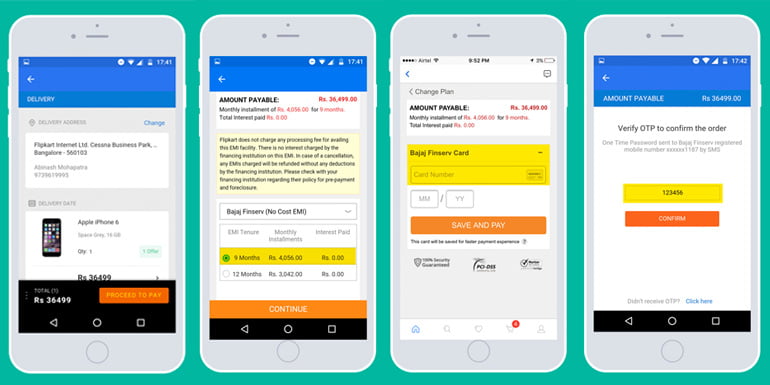This is a detailed caption for an image showing four side-by-side mobile application screenshots on a teal rectangle background:

The image showcases four side-by-side screenshots of a mobile application, each displayed within a gray, emulated smartphone frame. These screenshots are set against a teal rectangle background. The application appears to be an e-commerce platform, possibly focused on purchasing mobile phones.

- **First Screenshot**: Features a blue header at the top, followed by a central white section containing text. Below this is another white section displaying an image of a phone, suggesting a product listing. It includes a pricing section in an unspecified currency and an orange button labeled "Proceed to Pay."

- **Second Screenshot**: Also starts with a blue header, followed by a white section that displays the amount payable. Below this, a yellow section likely contains terms and conditions. The bottom part features payment terms highlighted in yellow, concluding with an orange button labeled "Continue."

- **Third Screenshot**: This one reaffirms the amount payable in a white section at the top. The central yellow section now includes fields for entering credit card details, such as the card number and expiration date. There is also an option to "Save and Pay" at the bottom, indicated by the orange button.

- **Fourth Screenshot**: This screen prompts the user to enter a one-time PIN code to confirm the purchase. The code entry field is highlighted in yellow, and the interface concludes with an orange "Confirm" button.

Overall, the sequential flow in the screenshots suggests the step-by-step process of purchasing a phone through the mobile application.